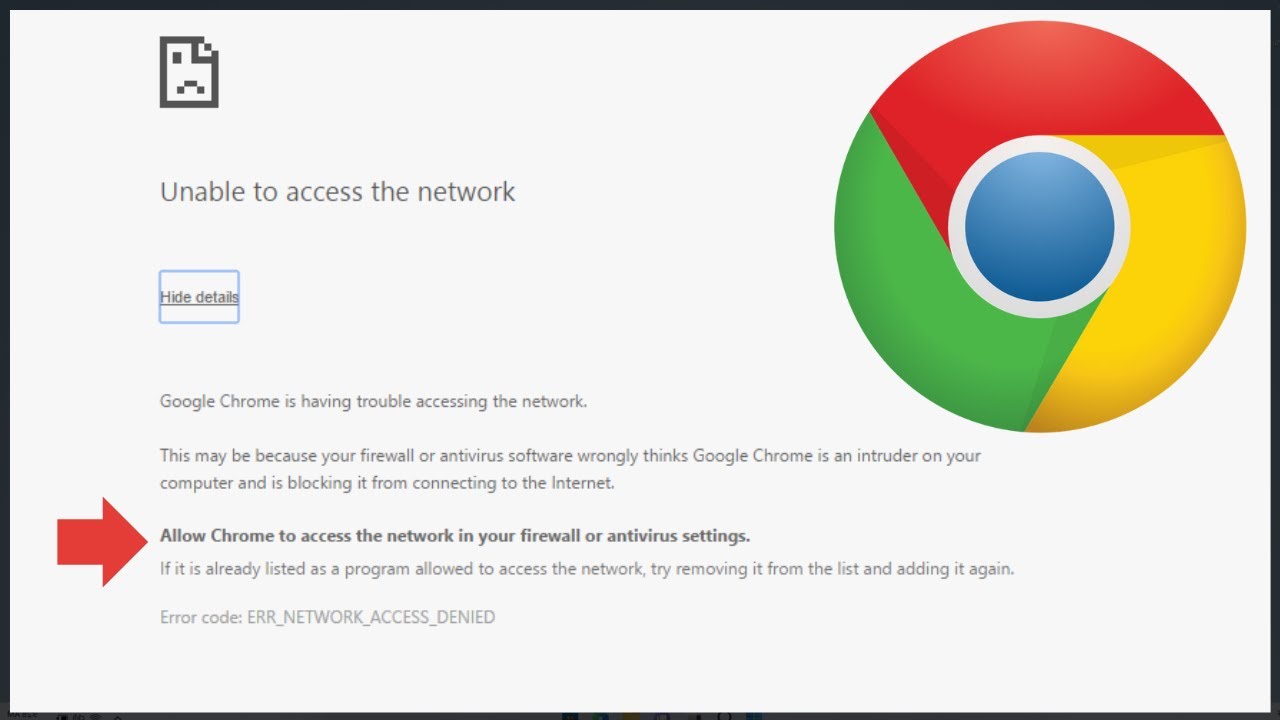In this screenshot of a Google site, a horizontally elongated rectangular black border encompasses a white background. Dominating the upper right corner is the standard Google Chrome icon, showcasing its distinctive colors: red, yellow, and green, with a blue circle in the center. In the upper left corner, a gray message reads, "Unable to access the network." Directly below this, a "Hide details" link appears in black text, outlined in blue. Underneath this link, additional gray text states, "Google Chrome is having trouble accessing the network." There is a prominent, bold red arrow pointing to the right towards a crucial message: "Allow Chrome to access the networks in your firewall or antivirus settings."